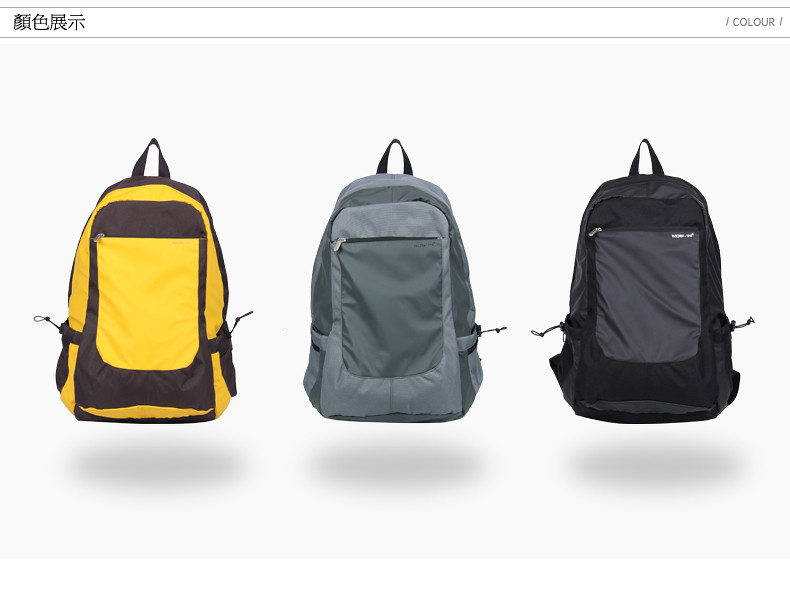This picture showcases three sturdy canvas backpacks, each suspended against a clean white background, casting subtle gray shadows beneath them. In the top left corner of the image, three black characters in an Asian language are visible, while the upper right corner features the word "colour" flanked by forward slashes, both bordered by thin horizontal lines. 

Starting from the left, the first backpack is a vibrant yellow with deep brown accents, featuring a black handle and a prominent yellow front zipper. The middle backpack is a blend of light and dark gray tones, with a gray handle and a darker gray front zipper area. Lastly, the backpack on the right is mainly black with a lighter, almost washed-out gray pocket, and a black handle. Each backpack is upright, facing the camera, with handles positioned as if ready to be hung in a locker or carried.